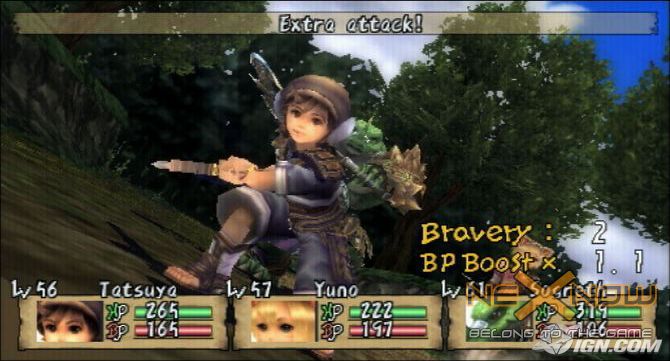The image shows a still from a computer game featuring a young female character, likely Tatsuya, dressed in medieval or hunting gear. She is crouched down, partially turned away from the camera, holding a knife or spear in her left hand, with a small green creature on her back. The setting is a detailed forest scene, with brown ground, blue sky partially visible, and tree lines covering most of the background along with some white clouds. The top of the screen displays "extra attack" in a header bar. At the bottom, game stats are shown, including bravery level BP boost at 1.1 and the names and stats of three players: Tatsuya, Yuno, and Susreth. The image also features score or power indicators as red and green bars next to each player's avatar. This appears to be a screenshot of friends engaging in an online competitive game, with Tatsuya being the character depicted in the main image.